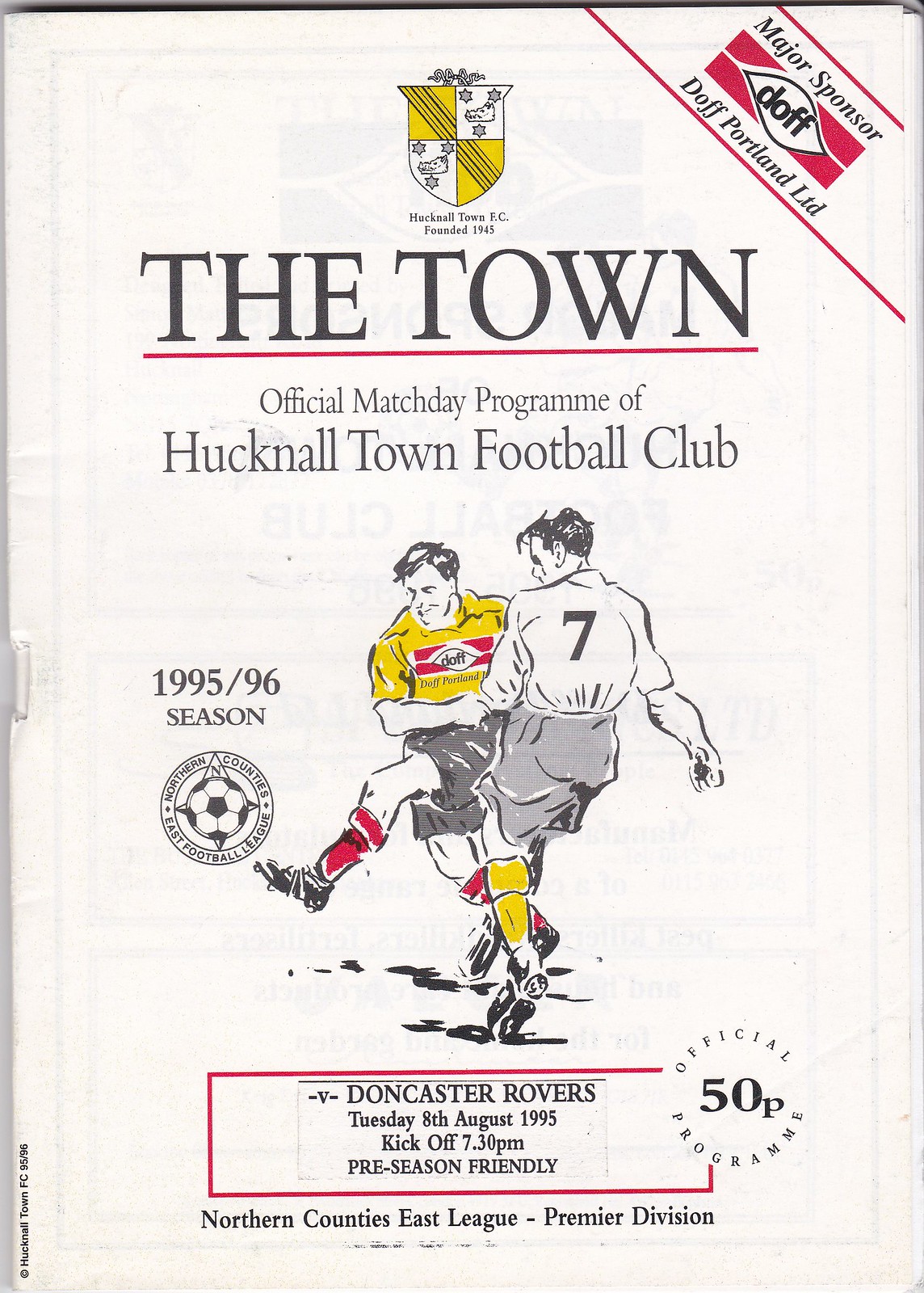The image is a vintage pamphlet cover for a football match, with a pinkish hue. It prominently displays the title "The Town" in bold, black, underlined text at the top center. Above this, there's a shield insignia in yellow and black, with "Hucknall Town FC, founded 1945" at the topmost part of the pamphlet. The top left corner features a sponsor's mention: "Major Sponsor Doff, Doff Portland LTD."

Directly below the title, the pamphlet states: "Official Match Day Program of Hucknall Town Football Club," signifying its purpose for match day. A central illustration showcases two footballers, one in a yellow jersey and the other in white, engaging with a soccer ball. The text wrapped around the soccer ball reads "Northern Counties East Football League."

The pamphlet marks the 1995-96 season above the illustration. At the bottom, there’s a red-outlined box with details about a preseason friendly match: "V. Doncaster Rovers, Tuesday, 8th August, 1995, kickoff, 7.30 p.m." Below this box, it specifie,s "Northern Counties East League, Premier Division." On the right side, a small circle reads "Official Program 50P." The entire design is classic of a football club program, reflecting Hucknall Town Football Club’s heritage and match details.